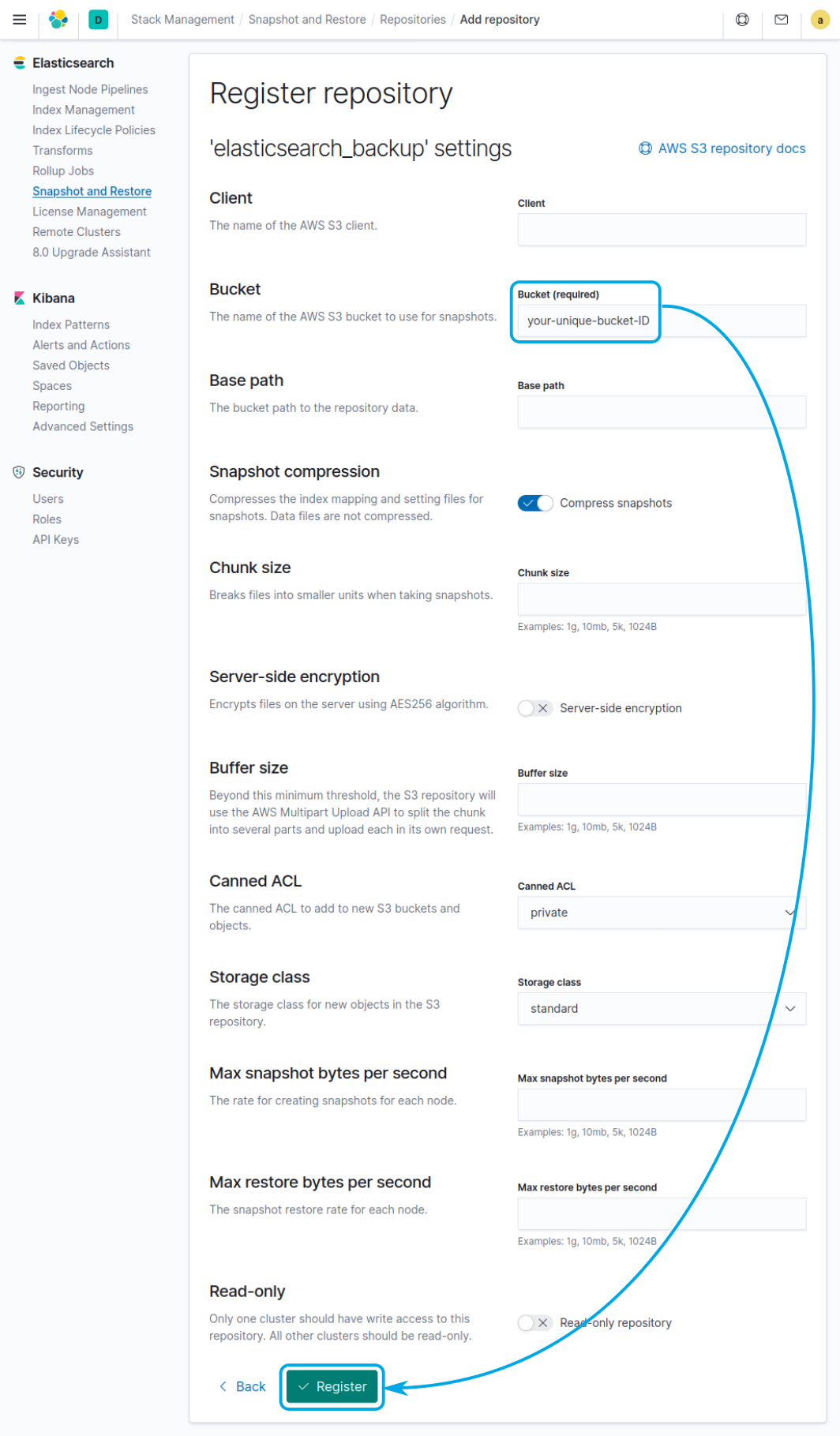The image depicts a highly detailed and technical page from a software development site, focusing on stack management and snapshot functionalities. The section displayed is titled "Register Repository," where users can add a new repository by filling out several text fields, including Client Name, Bucket ID, Base Path, and Snapshot Compression. Options like choosing whether to compress snapshots, setting Chunk Size, enabling Server Side Encryption, configuring Buffer Size, and setting Canned ACLs are available. This advanced interface is geared towards experienced users well-versed in such technical details.

On the left side of the page, there's a navigation pane with three main subsections: Elasticsearch, Kibana, and Security. The Security section includes options for Users, Roles, and API Keys. Additionally, the presence of Amazon Web Services (AWS) branding in the top right corner suggests that this page is part of a larger AWS-integrated platform.